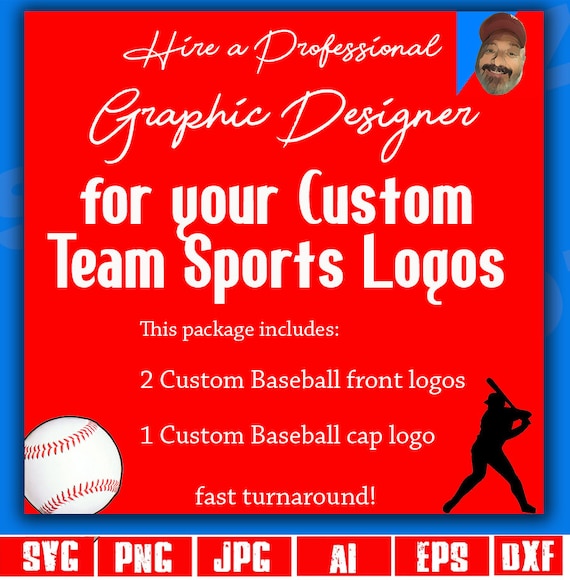The advertisement features a vibrant red background framed by a blue border. At the top, a photograph of a bearded man wearing a baseball cap introduces the ad. In elegant cursive writing, it reads "Hire a Professional," followed by "Graphic Designer" in bold print. Below, the ad continues with "for your custom team sports logos." 

In thin white print, the ad details what the package includes: "Two custom baseball front logos, one custom baseball cap logo, fast turnaround." A white and red baseball sits in the bottom left corner, while the silhouette of a baseball batter occupies the right bottom corner. Additionally, a block of six red sections at the bottom showcases various file formats available: SVG, PNG, JPG, AI, EPS, and DXF.